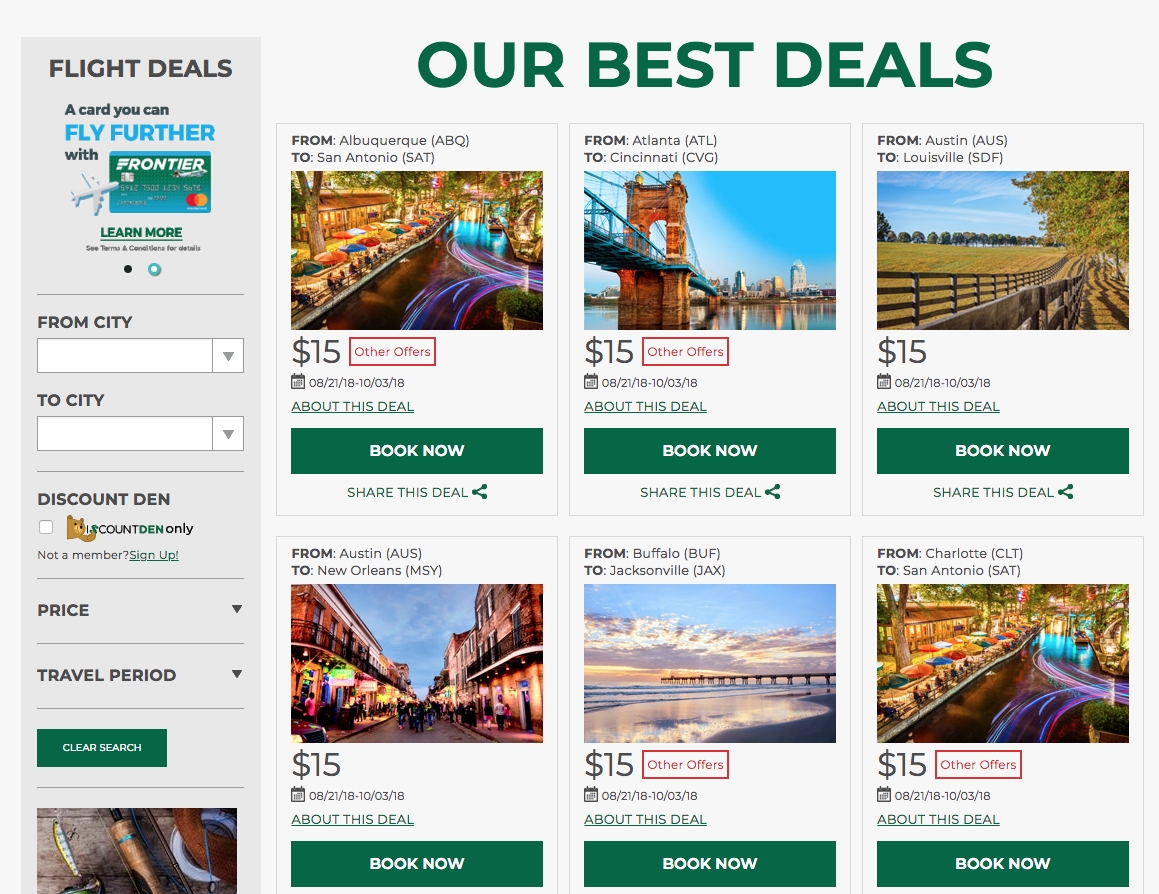The image shows a booking website dedicated to providing deals on flights, primarily featuring Frontier Airlines. At the top of the page, a prominent banner reads "Our Best Deals." On the left side of the site, there is a menu labeled "Flight Details," where users can presumably input and search for specific flight information.

The main section of the website displays six distinct promotional boxes, each showcasing a flight deal with vibrant images of the respective destinations. 

1. **Albuquerque to San Antonio**
2. **Atlantis to Cincinnati**
3. **Austin to Louisville**
4. **Austin to New Orleans** - spotlighting a remarkable deal for $15
5. **Buffalo to Jacksonville**
6. **Charlotte to San Antonio**

Each of these boxes features a green "Book Now" button, encouraging immediate booking of the highlighted flights. Additionally, there is text indicating that Frontier Airlines is offering these deals, with slogans like "You can fly further" scattered throughout. The left sidebar has options for selecting the departure and destination cities, facilitating a user-friendly booking experience for shorter flights.